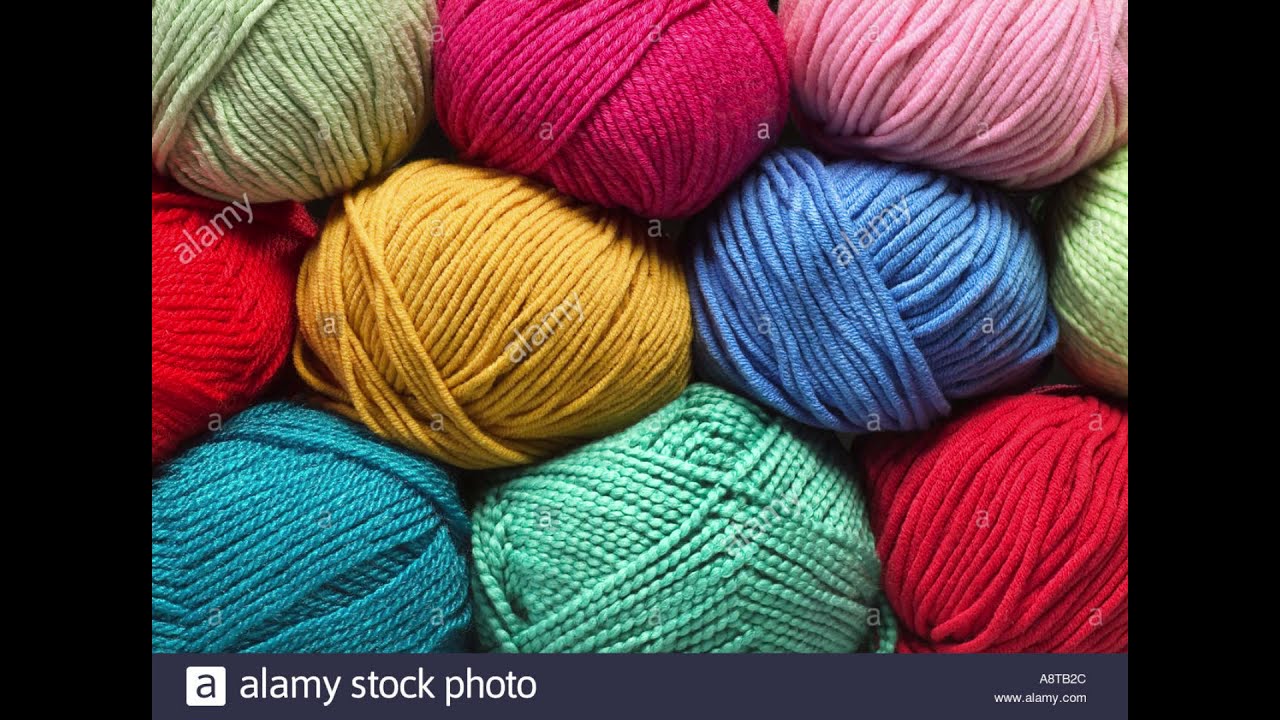This vibrant, detailed photo showcases a carefully arranged collection of various yarn balls, each exuding a distinct color and texture. The image is organized into three rows: the top row features a minty green ball in the top left corner, followed by a magenta ball in the center, and a light pink ball on the top right. The middle row presents a reddish orange ball, flanked by a yellow ball and a blue ball, with another minty green ball next to them. The bottom row includes a blue ball, a teal ball, and a red ball of yarn. The photo is heavily watermarked, with the text "Alamy Stock Photo" prominently displayed at the bottom, along with the website "alamy.com" and accompanying details. The watermark, which incorporates a lowercase "a" in a white box, runs diagonally across the image, ensuring the source is unmistakable. This meticulous arrangement and watermarking hint at its professional use, ensuring the image's protection from unauthorized usage.